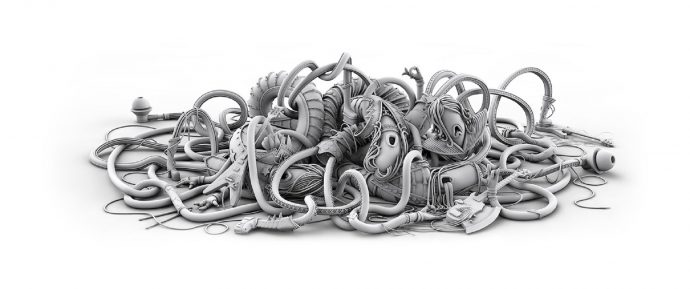The image portrays a detailed grayscale digital rendering on a completely white background, depicting a chaotic jumble of various objects. Among the indistinguishable mess of cables, ropes, and wires, some items distinctly emerge. Interspersed within the tangled web, there are guitars—some intact while others are broken—as well as drumsticks. Snake-like figures with occasional features like eyes and mouths weave through the clutter, adding to the intricate confusion. Earbuds are scattered among these items. Despite the lack of color, the high-detail 3D artwork highlights the complexity and intentional disarray, leaving an ambiguous interpretation of its purpose or origin.